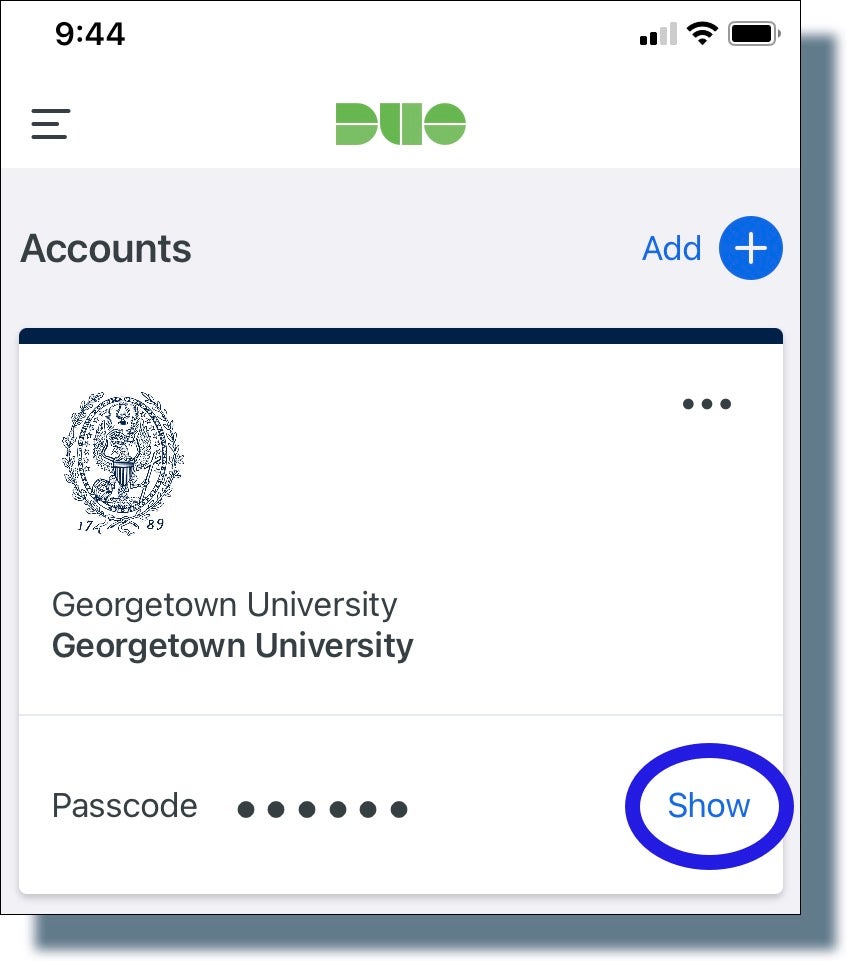The image showcases a smartphone screen displaying an application page for "JOOL." At the top center, "JOOL" is prominently written in green text against a white background. The top left corner features a black menu icon, represented by three horizontal lines. 

Beneath "JOOL," the background transitions to gray where the word "accounts" is displayed on the left. Opposite to this, on the right side, there is a blue button labeled "ETH," accompanied by a blue-shaded circle containing a white plus sign.

Directly below this, "Georgetown University" is written twice; the first instance is in regular black text, while the second is bold. Above the text on the left is the Georgetown University logo in blue, matching the white background of the page.

On the left side, there is a main option icon featuring three black, horizontal dots. Beneath the university text, the word "passcode" is displayed with six concealed dots to the right, indicating the hidden passcode. On the right side, next to the passcode, there is another blue button labeled "show," encircled by a blue border. This button is intended to reveal the passcode when pressed.